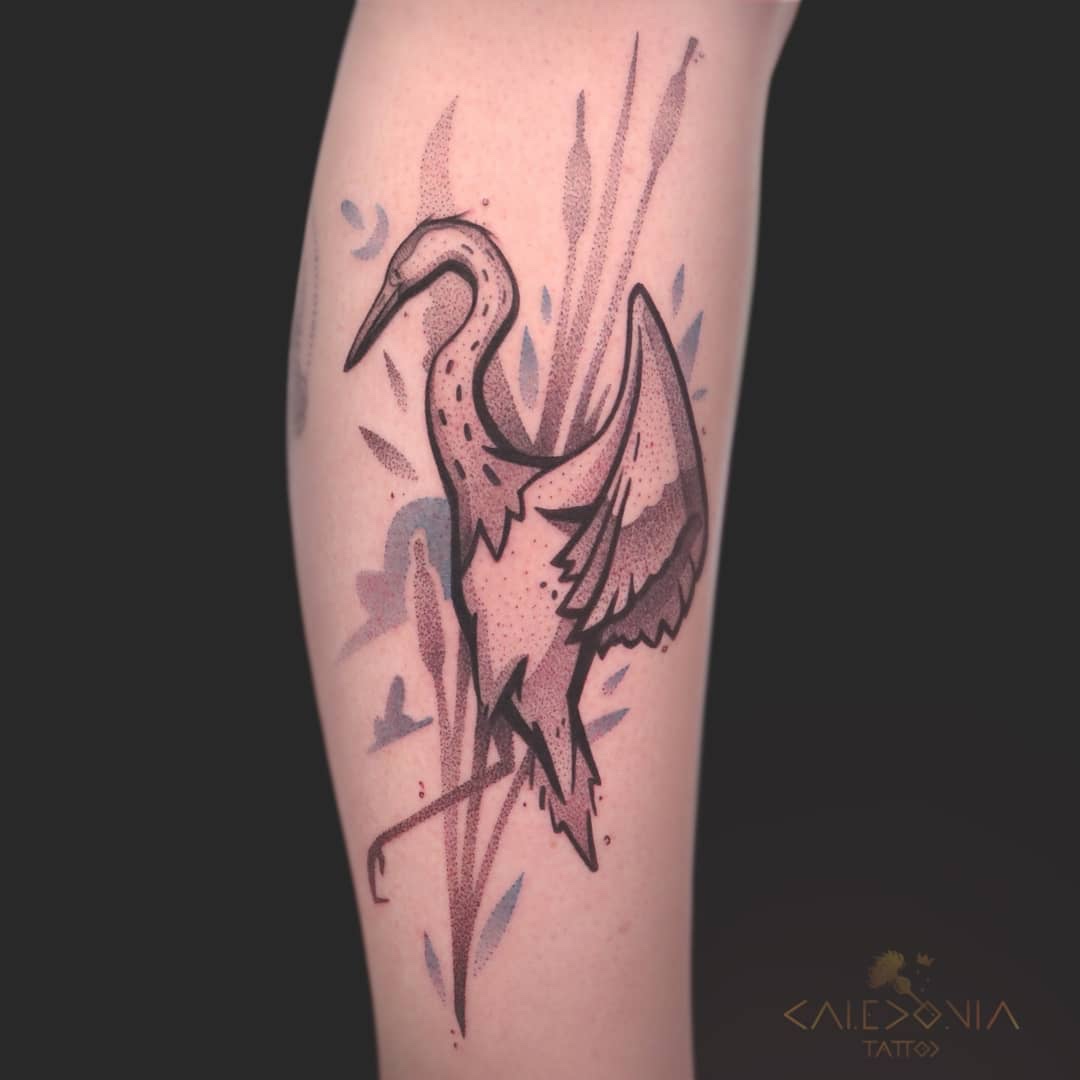This color photograph displays a close-up view of a pale, fair-skinned person's arm featuring a detailed tattoo of a crane or great blue heron. The tattoo is showcased against a black background, with two black panels that emphasize the arm. The stylized bird, primarily in shades of white, brown, and black with touches of pink and blue, stands with one leg raised and its wing slightly lifted. The bird's long neck is adorned with black speckles, and it has a prominent beak and feathered cap. Behind the bird, a shaded background reveals a cluster of cattails and clouds, contributing to a slightly cartoonish, yet intricate design. Additional elements include pink or reddish reeds and splashes of water, creating a sense of motion. The detailed feathering on the crane, especially along its back and wings, gives a three-dimensional effect. The lower right corner of the image contains the text "Kaidonia Tattoo," stylized in Greek or ancient lettering, identifying the tattoo studio.